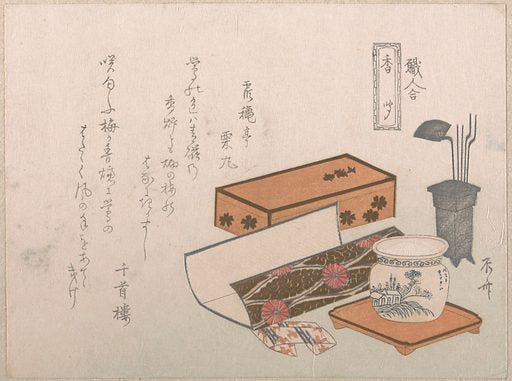This detailed drawing, rich in Japanese cultural elements, depicts a serene and organized setting featuring various traditional items. On the left side, Japanese characters are artistically inscribed from top to bottom. Central to the arrangement is a rectangular wooden box adorned with black floral designs. In front of the box lies a piece of beautifully folded paper, possibly origami, designed with intricate black fish scales and vibrant red poppy flowers. To the right of the box, there rests a small tan vase embellished with an illustration of a house amidst bluish-green grass and bushes, also featuring Japanese script. Positioned behind these elements is a calligraphy container, holding several brush-like instruments; two of which are straight rods, while the others curve before straightening out again. These traditional implements are complemented by a fanned-out brush on the left side. The scene exudes a vintage aesthetic, drawing viewers into its tranquil, meticulously composed atmosphere.